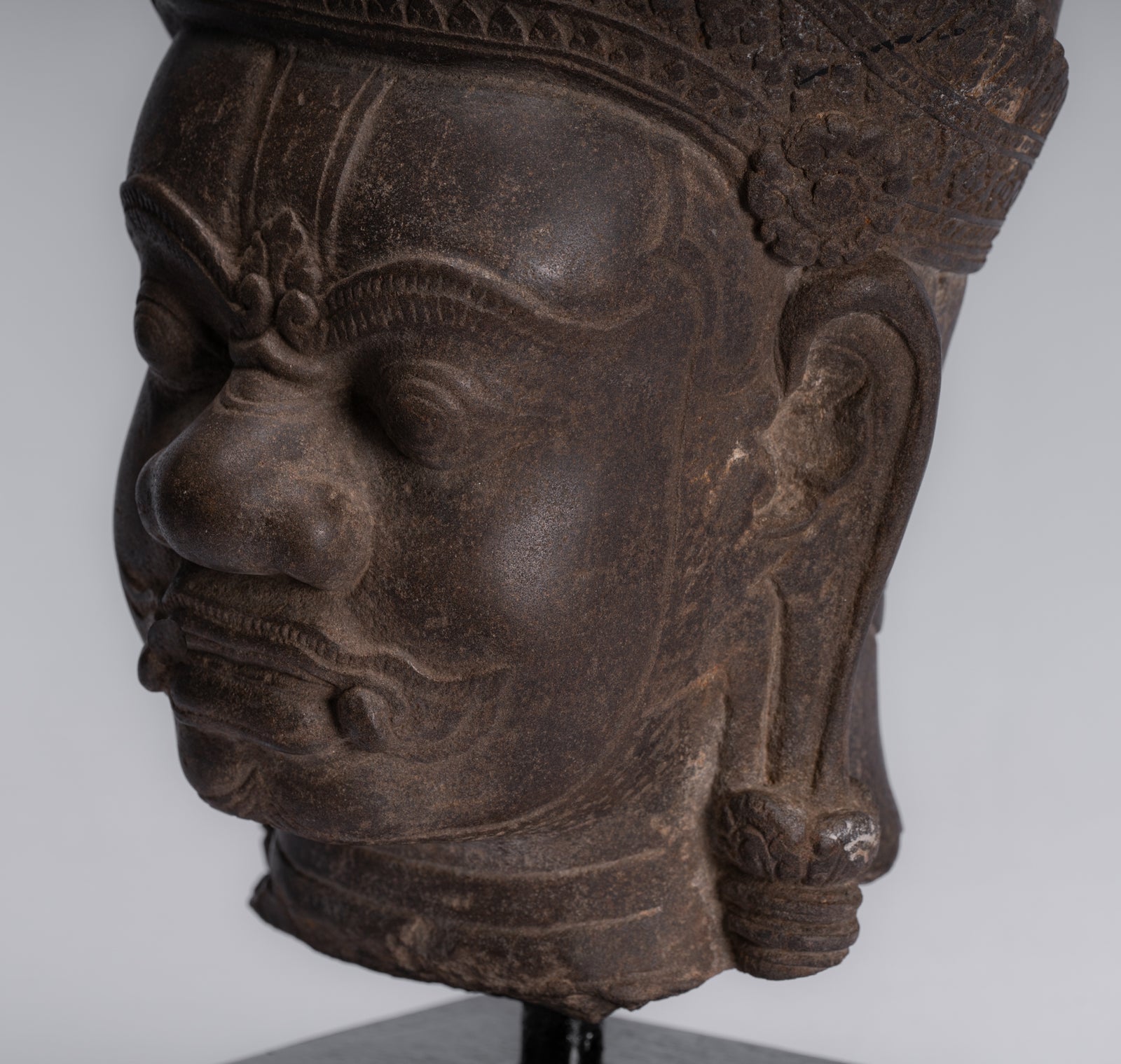This detailed close-up image captures a large, ancient-looking head sculpture that appears museum or library-worthy, but could also be a statement piece in a home. The sculpture, which seems to be made from copper or cast iron with a rich brown or copper tone, has a finely etched surface giving it an antiquated, Indiana Jones-esque feel. It showcases a single, colossal head adorned with a headdress or crown that includes circular, flower-like details near the ears. The facial features are exaggerated, with prominent, wide eyes, a notably large nose and mouth, and big cheeks. The head, facing slightly to the left, appears massive and heavy, possibly indicating its representation of a king or a significant figure. The piece is remarkably well-preserved, displaying minimal rust or discoloration. The elongated ears hint at cultural or historical significance, accented further by the small tusks emerging from each side of the mouth and a long necklace hanging from the ears.